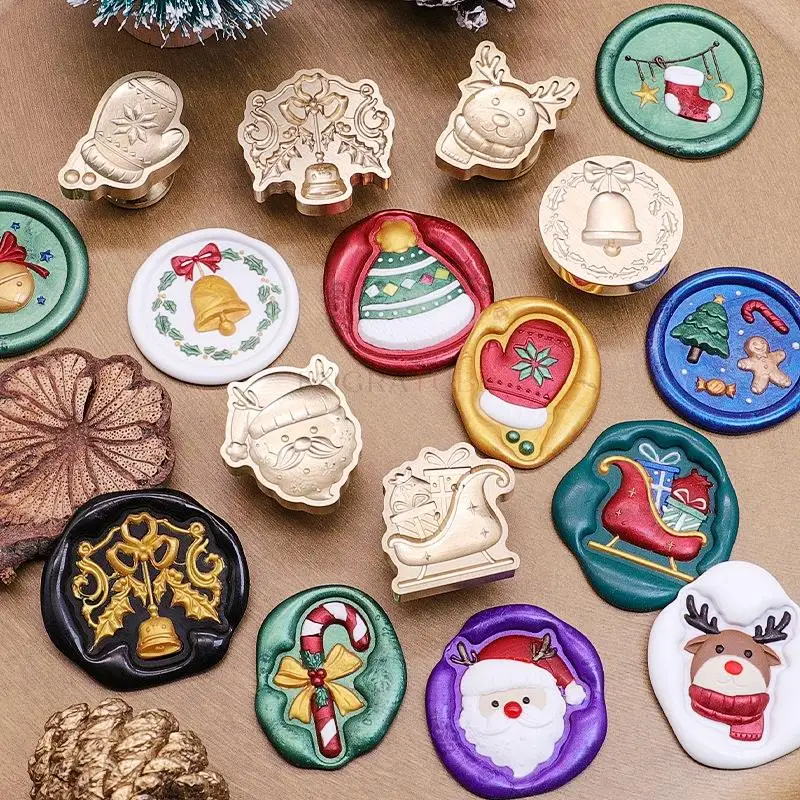The vertical, full-color photograph showcases a meticulously staged indoor scene, likely illuminated by natural light. Displayed against a plain, brown tabletop, the image features an array of exquisitely hand-painted Christmas ornaments, each made from baked clay. The ornaments are meticulously detailed, presenting a vibrant palette of red, green, gold, blue, and black.

The top row includes gold-painted designs like mittens, a reindeer, and a bell adorned with leaves. Adjacent to these, a green-painted ornament showcases a Christmas stocking, a crescent moon, and a star. The second row features a continuation of the festive theme, with green ornaments depicting stars and Christmas balls, alongside a white ornament with a bell and a white-and-red ornament showcasing a hat. Another gold bell ornament completes the set.

Further down, the collection includes a variety of shapes and colors: a brown flower, a gold Santa Claus, a red mitten bordered in gold, and a circular blue ornament embellished with a tree, a gingerbread boy, candy canes, and candies. Additional rows display similar Christmas motifs, including Santa Claus’s face, a reindeer, candy canes, a Christmas glove, and a sleigh, all vividly painted and ready to adorn a festive setting. The overall image is clear and brightly lit, capturing the intricate details and bright colors of the holiday decorations.